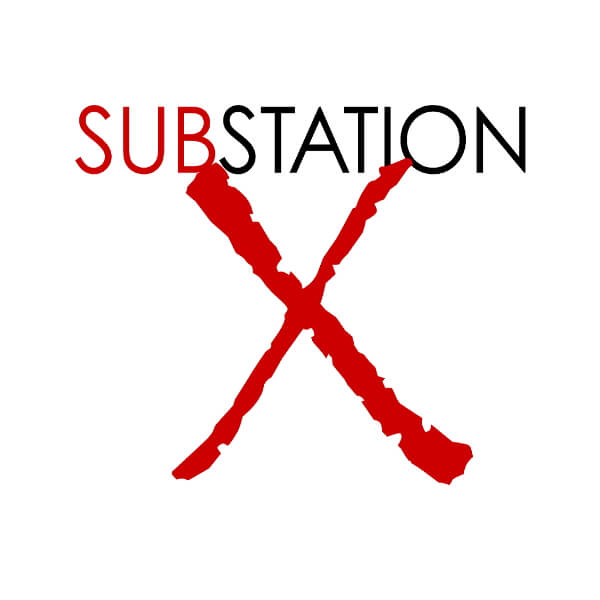The image features a minimalist design against a solid white background. Centered at the top is the word "SUBSTATION," with "SUB" in bold red capital letters and "STATION" in black capital letters. Beneath this text, taking up a significant portion of the image, is a large, jagged-edged red X with a distinctive uneven design. The X has a thicker diagonal stroke running from the upper left to the lower right and a thinner stroke crossing from the upper right to the lower left, with irregular edges and chunks missing, giving it a hacked or bitten appearance. The simplicity and graphic style of the image suggest it could be a company logo, a band or album cover, or promotional material for a product or game. There's no additional text, symbols, or references in the image.